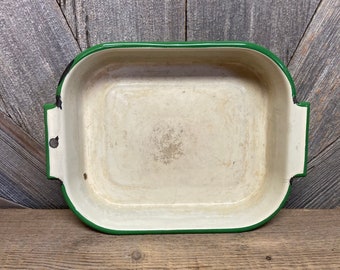The image shows an aged, cream-colored metal casserole dish or baking pan positioned on its side against a wooden wall. The wall's wooden planks are greyish in color and are placed diagonally, directing focus towards the dish. The dish, which features a green border, is marked with brownish-orange stains, indicating frequent use. The inside of the dish, which is fairly dingy, was initially white but is now discolored. The dish is resting on a dark brown wooden floor, with possible remnants of a sticker or a logo visible on the left handle and center. Leaning against the rustic wood-plank backdrop, the casserole dish’s scuffed and worn appearance gives it a character that suggests a history of extensive utility.